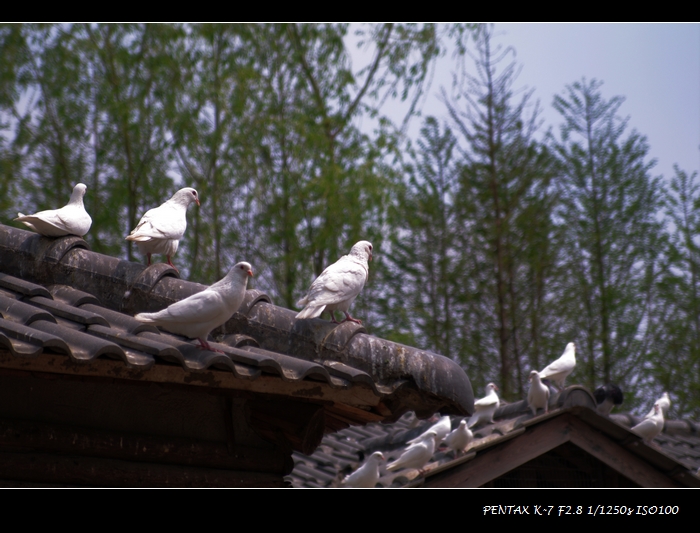The photograph, taken outdoors, captures a scene with a black tile roof that appears discolored, possibly covered in dirt, mildew, and bird droppings. The roof, which looks like that of a house or cabin, consists of two sections. The top section features four white pigeons with orange beaks, positioned in a staggered formation: one in the upper left, another below it, and two more in front of them. The lower section of the roof displays a row of five small white doves, along with three more white doves as you move towards the right-hand side. The background showcases a large row of tall, green, thin-trunked trees, and a bluish-gray, slightly overcast sky. The image is bordered at the top and bottom by a black strip with a thin white line. In the bottom right-hand corner, there is white text that reads, "Pentax K7 F2.8 1/1250 ISO 100."